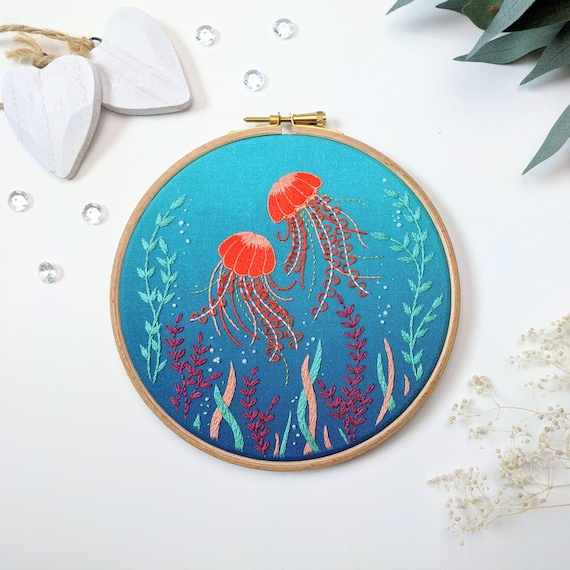In this detailed embroidery artwork, we see a meticulously done needlepoint depicting an underwater scene. The embroidery is held within a beige hoop with a gold-colored ring fastener at the top, ensuring a tight fit. The central focus features two red jellyfish, complete with intricate thin white lines and red squiggles representing their tentacles. Positioned diagonally, one jellyfish floats above on the right, while the other is situated to the left. Surrounding the jellyfish are delicate strings of green leaves, mimicking underwater flora, along with white embroidered dots that resemble bubbles.

On the top left, the piece includes two grayish-white hearts, each roughly a quarter-inch thick and a couple of inches tall, anchored by a rough white or beige string threaded through holes at the top of each heart. Additionally, the bottom of the embroidery showcases twisting blue and pink strands that add a dynamic element to the marine environment. The entire scene is stitched onto a blue fabric, making the vibrant colors of the jellyfish and plants stand out vividly. The artwork rests on a white table adorned with decor, complementing the detailed and vividly colored seabed tapestry.